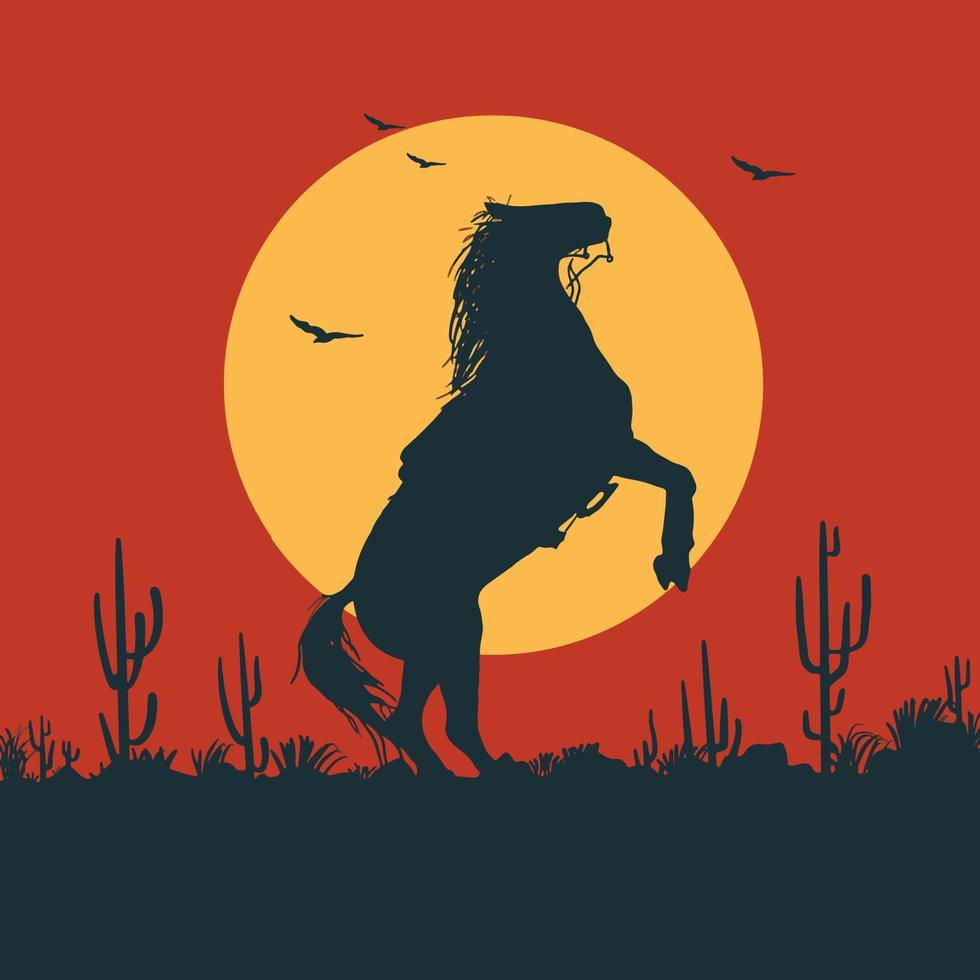The image is a detailed, computer-generated silhouette drawing or painting of a black horse rearing up on its hind legs, facing towards the right. The horse features a fluffy mane and a bridle, with part of its saddle visible. It is set against a reddish-brown backdrop dominated by a large, luminous yellow moon. Below the horse, the ground is depicted in black, adorned with silhouettes of cactus plants, enhancing the desert-like setting. Above the horse, four black silhouetted birds are seen flying. The entire composition emphasizes the stark contrast between the dark silhouettes and the vibrant colors of the sky and moon, accentuating the dramatic and wild atmosphere. There is no text on the image.